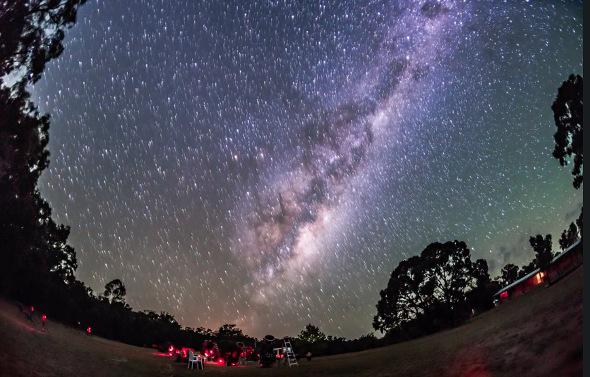The horizontally aligned, rectangular image portrays a clear, star-filled night sky likely free from light pollution. The sky is a blend of gray with a greenish tint near the horizon, sprinkled densely with white speckles representing stars, suggesting a view of the Milky Way galaxy. Among this celestial display, there's a notable diagonal cloud, brown mixed with white, stretching from the middle towards the upper part of the image, resembling a rock.

The ground below is portrayed with an arching contour, dipping down from the left, traversing the center, then rising upward towards the right. This land area is densely populated with trees from the left top corner, sweeping down across and then up again to the right, enveloping the scene. 

Central to the image, amidst this natural panorama, there's a gathering perhaps for a stargazing event. Red lights suggestive of car headlights and possible campfires or tents hint at people camping or stationed there, possibly in lawn chairs, gazing up at the cosmic spectacle. A couple of indistinct structures, possibly houses, add to the scene. The image, captured at night, is a wide-angle shot that encapsulates the vast, awe-inspiring view of a galaxy-studded night sky and the serene, tree-lined land below.